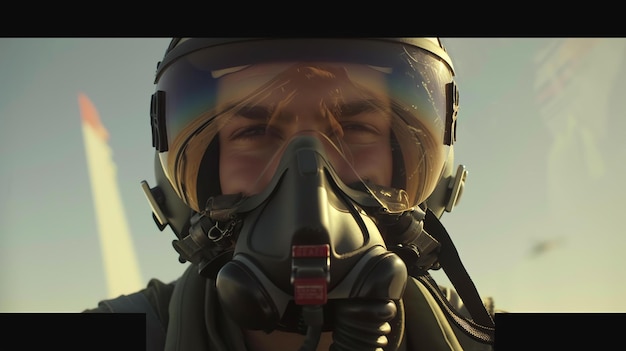This horizontal rectangular image is a close-up of a pilot, possibly Tom Cruise as portrayed in Top Gun Maverick, taken from inside the cockpit of an aircraft. The pilot's head and upper shoulders are prominently featured, framed by black letterboxing bars at the top and bottom of the image, with the bottom bar broken in the middle. The background consists of a light blue sky, slightly darker on the left side, with a faint exhaust streak and a pink object resembling a missile or airplane in the upper left quadrant.

The pilot, wearing a gray helmet with a clear visor, dons a face mask and goggles. The triangular oxygen mask, gray in color, covers the lower half of his face, with a tube extending from the right side. His eyes, forehead, and part of his cheeks are visible through the goggles and above the mask, accentuated by a hint of his eyebrows. Over his ears, the helmet snugly fits, hinting at the intense environment of a fighter jet. The background also shows the tail of an airplane over his shoulder, enhancing the aviation context.